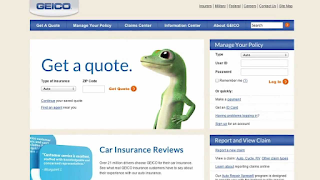**Detailed Description of GEICO Website Screenshot:**

The screenshot showcases the GEICO website with a tan background. In the top left corner, the prominent GEICO logo is displayed in blue, all capital letters set against a silver shield-like background. Beneath the logo, multiple tabs are visible within a blue rectangular bar. The tabs, though hard to read due to blurriness, include options like "Get a Quote," "Manage Your Policy," and "Claims Center." At the top, a thin blue bar spans across with a search option positioned on the right.

Below these navigation tabs, there’s a primary section for obtaining a quote, featuring fields to input your zip code and car details. Dominating this section is an image of the recognizable GEICO gecko. Adjacent to the gecko, on the upper right side of the page, the "Manage Your Policy" option is indicated for users to enter their information. Beneath it, another section allows users to report and view claims, located at the bottom right side of the screen, with several links for easy navigation.

Despite the overall blurriness, the screenshot clearly outlines various functionalities available on the GEICO website, such as getting quotes, managing policies, and reporting claims.